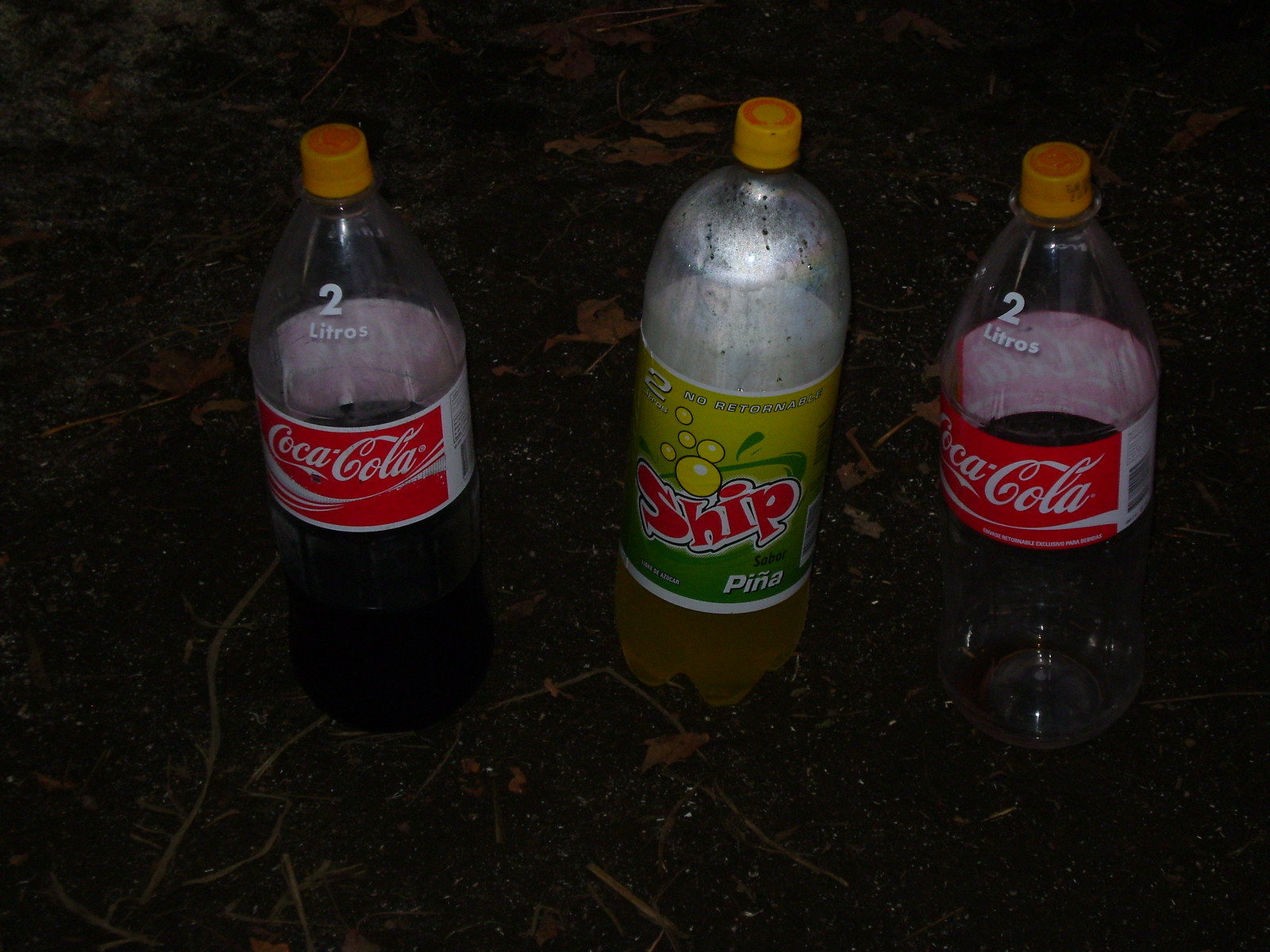This is a photograph of three two-liter bottles of soda taken in a dimly lit, nighttime outdoor setting. The poor quality of the image makes it challenging to discern certain details clearly. The central bottle is a South American soft drink called "Ship," with a green label featuring red lettering, and it is labeled "Sabor Piña" with a yellow cap. On either side of this bottle are two two-liter Coca-Cola bottles, each with yellow caps. One of the Coca-Cola bottles appears to be completely empty, while the other has about a third of its contents remaining. The bottles seem to be placed on a surface that resembles wet leaves and sticks, suggesting an outdoor environment, though the darkness makes it difficult to confirm. The overall ambient lighting, possibly from a camera flash, adds to the dim and dark quality of the photograph.